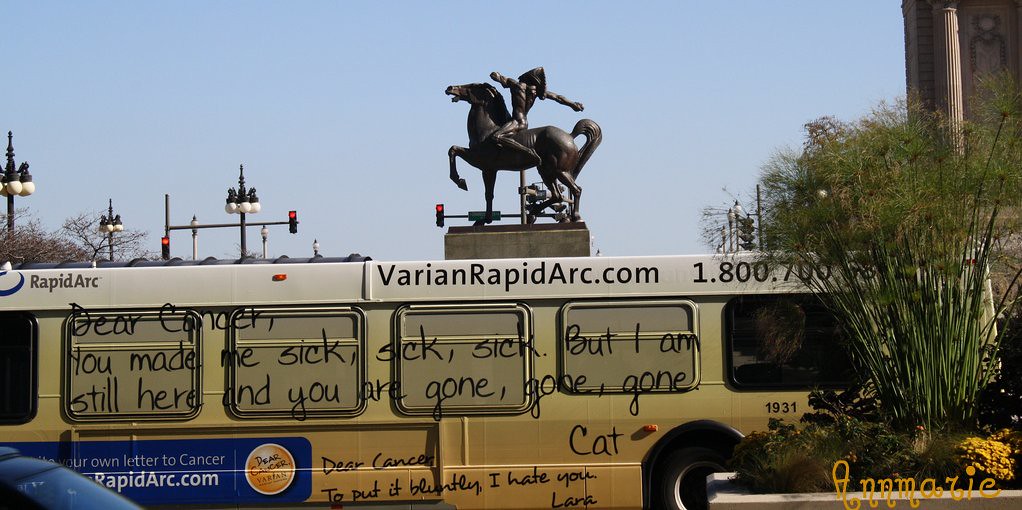The photograph captures a long bus prominently displayed in the bottom half of the image, extending off the left side and showcasing its front end on the right, partially obscured by a large plant with flowers in a raised planter. The bus has six windows, four of which have shades pulled down with black writing over them. The top of the bus displays the website "VarianRapidArc.com" along with a partially obscured phone number. On the side, there is an advertisement featuring the message: "Dear Cancer, you made me sick, sick, sick, but I am still here and you are gone, gone, gone. Dear Cancer, to put it bluntly, I hate you, Laura. Write your own letter to Cancer at RapidArc.com." This message is accompanied by a blue background and yellow writing. Behind the bus, an imposing statue of a man on a horse, pointing to the left and mounted on a pedestal, dominates the background. The scene is set outdoors under a clear blue sky, with visible street lights, traffic lights, and a tall building to the right.